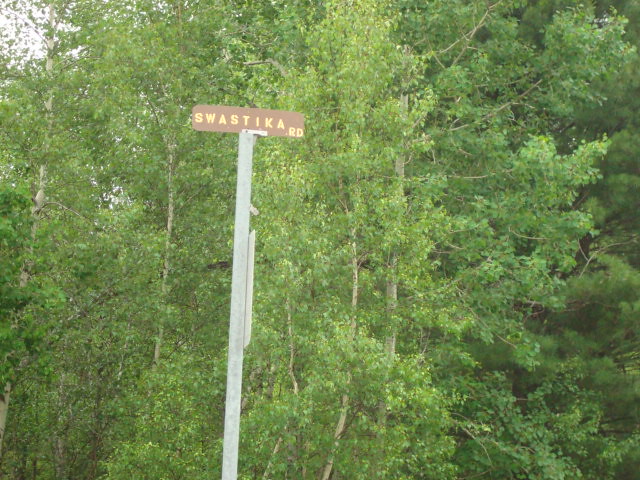In an outdoor photo capturing a lush, verdant landscape, dense green foliage envelopes the background with an assortment of trees in varying shades of green, indicating diverse types of foliage and the season being spring or summer. The sky behind the trees is brightly illuminated, reflecting a more whitish hue rather than a clear blue. Prominently in the foreground stands a signpost with a red sign displaying yellow letters that read "Swastika Road," an intriguing and unusual name for a street. Another sign is affixed to the pole but faces the opposite direction, its content obscured from view.